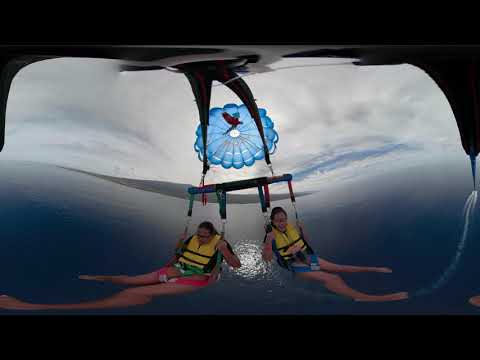The image captures a thrilling scene of two females parasailing over a dark, shadowed body of water on a cloudy day. The women are suspended by harnesses and yellow life vests, suggesting they are prepared for safety while engaging in this airborne adventure. Their legs dangle freely, indicating they are airborne and possibly just above the water's surface. Attached to a colorful parasail adorned with an eagle and a prominent hole in its center, they are part of a larger group participating in this activity; another blue parasail can be seen in the background against the cloudy sky. Patches of blue sky peek through the clouds, adding depth to the scene. The image itself appears slightly distorted, possibly due to lens effects or stretching, with black bars outlining the top. In the distant background, a faint, distorted mountain or hill appears on the horizon.